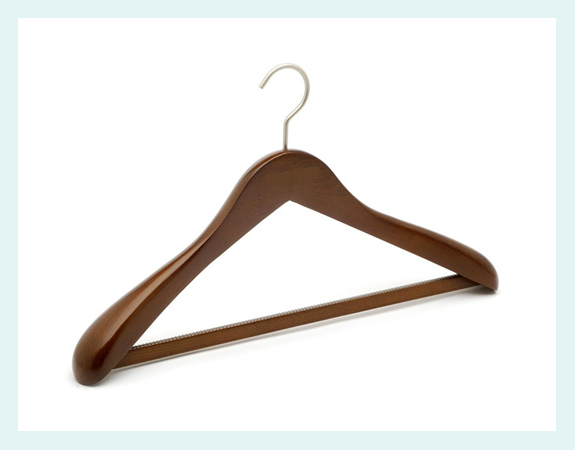The image features a straightforward composition with a white background framed by a thin, translucent, light blue border. At the center of the image is a detailed depiction of a wooden hanger. The hanger is crafted from a rich, medium to dark brown, glossy wood that has been lacquered to give it a shiny finish. The design includes rounded edges and a somewhat thicker body, suggesting it is suitable for hanging heavier items, such as coats or suits. The hanger is equipped with a metal hook at the top, which is shiny silver and curves to the left. Additionally, a wooden bar spans the bottom of the hanger, forming a triangular shape that provides an extra layer for hanging pants or other items.